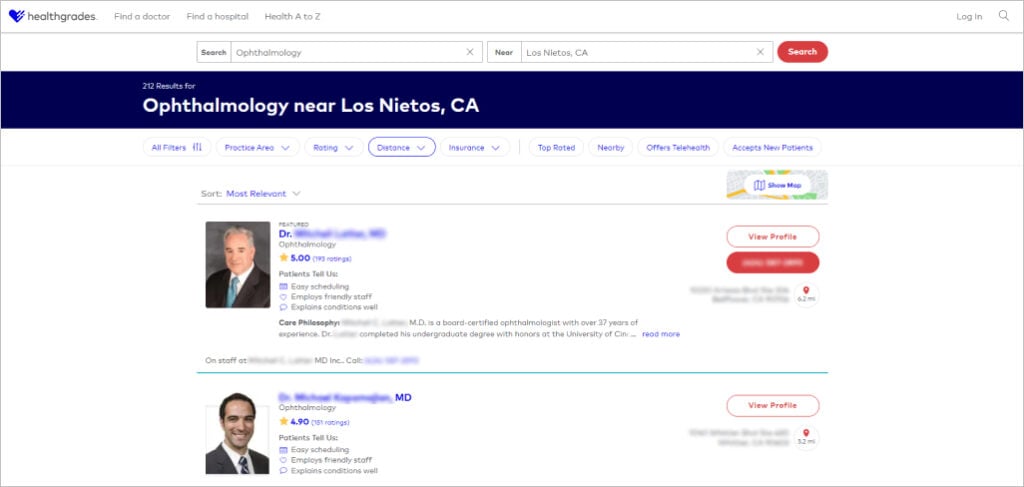### Detailed Caption

This is a screenshot of a healthcare website dedicated to providing health grades and information about medical professionals and facilities. Prominently displayed on the right-hand side are navigation options: "Find a Doctor," "Find a Hospital," and "Health A to Z." Just below these options is a login button, and next to it is a magnifying glass icon indicating a search feature for user inquiries.

Underneath these elements is a search bar currently populated with "ophthalmology" and set to the location "Los Nietos, California." The search results page lists potential ophthalmologists in and around Los Nietos, CA.

The search results can be refined using several filters located on the page, including options such as practice area, rating, distance (with the selected filter being "distance"), and insurance acceptance. Additional filter options include "Top Rated Only," "Nearby," "Offers Telehealth," and "Accepts New Patients."

For each listed doctor, there is basic information provided along with user ratings. In this particular view, only two doctors are shown. Each listing includes a brief overview of the doctor's credentials and practice information, along with an option to view their detailed profile for more comprehensive information.